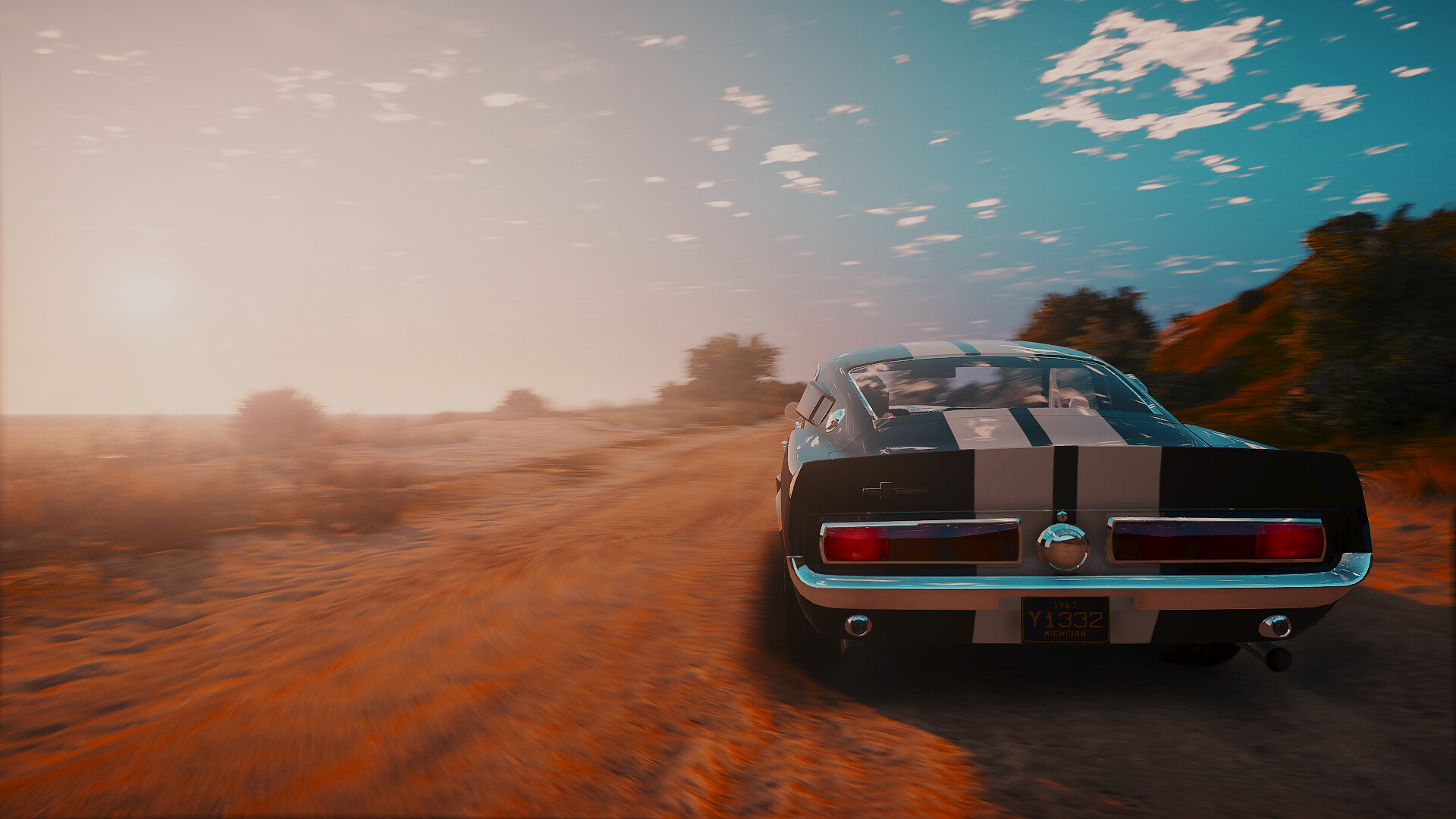The image captures an old classic race car driving down a rusty orange dirt road, possibly in a desert or countryside setting. The car, which is either dark blue or black, features two thick white stripes running from the back to the front, accentuating its sleek design. The focus is on the rear and top of the car as it drives away, revealing its red taillights, chrome exhaust pipes, and a blue license plate with yellow letters, although the text is not entirely legible. Through the rear window, the silhouette of a driver’s head is just visible. The surroundings include scattered bushes and trees, with a flat area on the left and a hill on the right. The sky above is a clear blue with a few white clouds, suggesting it is daytime. The setting exudes a sense of motion and adventure, enhanced by the hazy, bright light overlaying parts of the image.